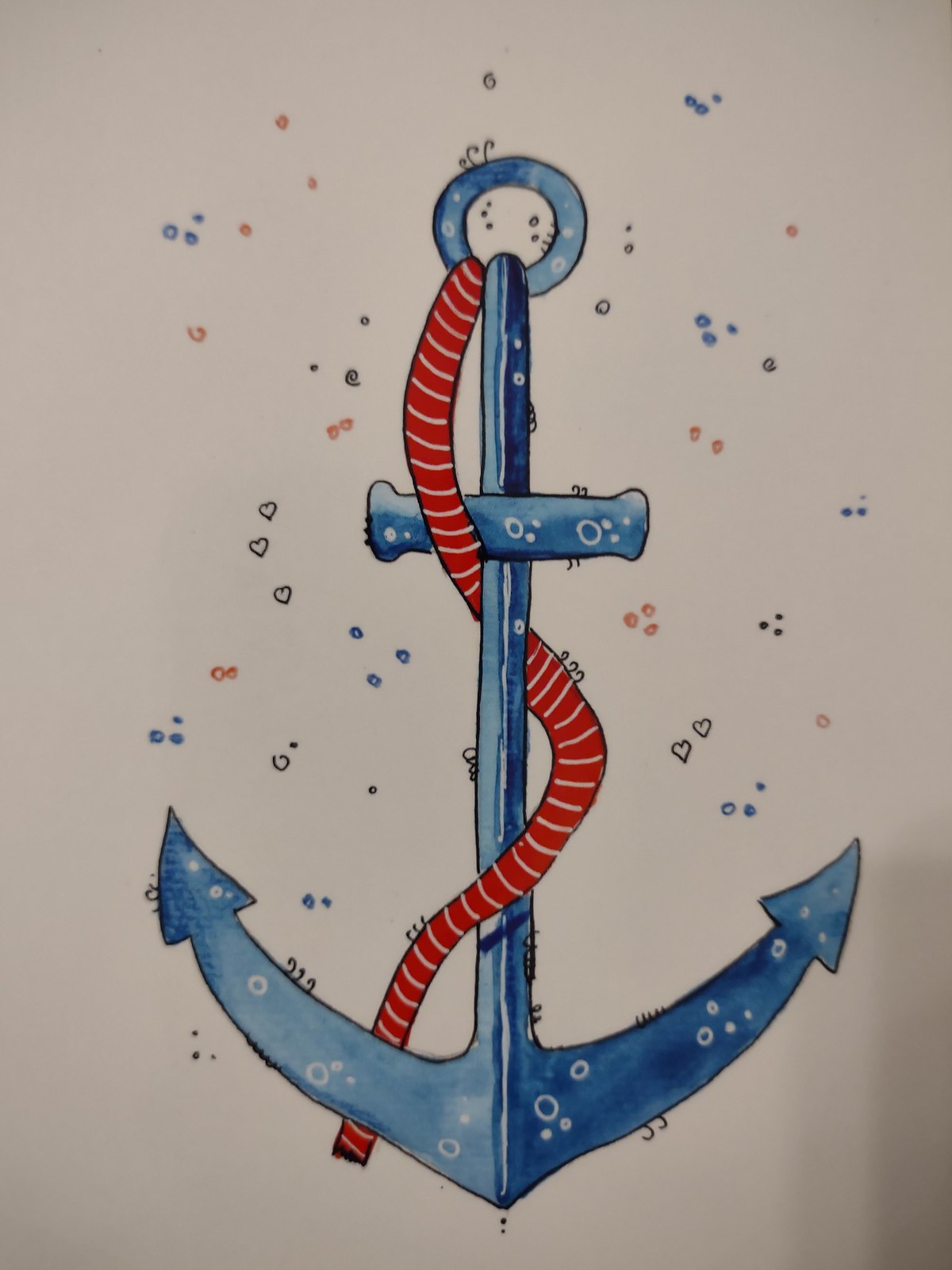The illustration depicts a detailed drawing of a blue boat anchor with a red-and-white striped rope attached to it. The anchor features a circular eyelet at the top, connected to another solid metal eyelet that extends straight down. Just below the top eyelet, a short horizontal bar crosses the anchor from left to right. The main body of the anchor gradually narrows as it curves outward on both sides, ending in pointed tips designed to dig into the seabed. Surrounding the anchor are small blue, white, and red circles, likely representing bubbles. The descriptive elements of the drawing highlight the functionality of the anchor, including how it is dropped into the water and secures itself to halt the boat's movement.